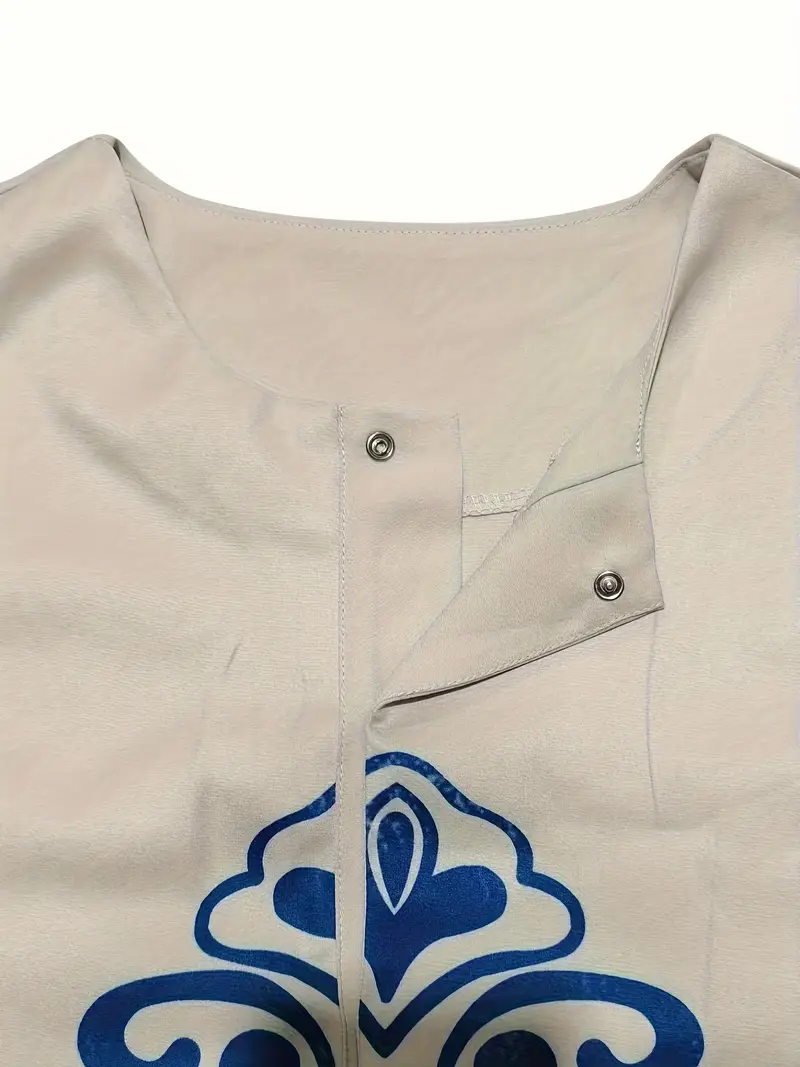A detailed close-up image captures the top half of a shirt, focusing primarily on the collar area. The shirt features a pair of snap buttons prominently positioned just beneath the collar, with one button's front side and the other's back side both visible, showcasing the male and female components of the snaps. The collar itself is slightly turned in on the right side of the image, providing a clear view of the backside of one snap button. A partial blue design is also noticeable on the shirt, though much of it is obscured due to the close proximity of the shot. The surrounding fabric can be seen extending to both the right and left sides of the collar.